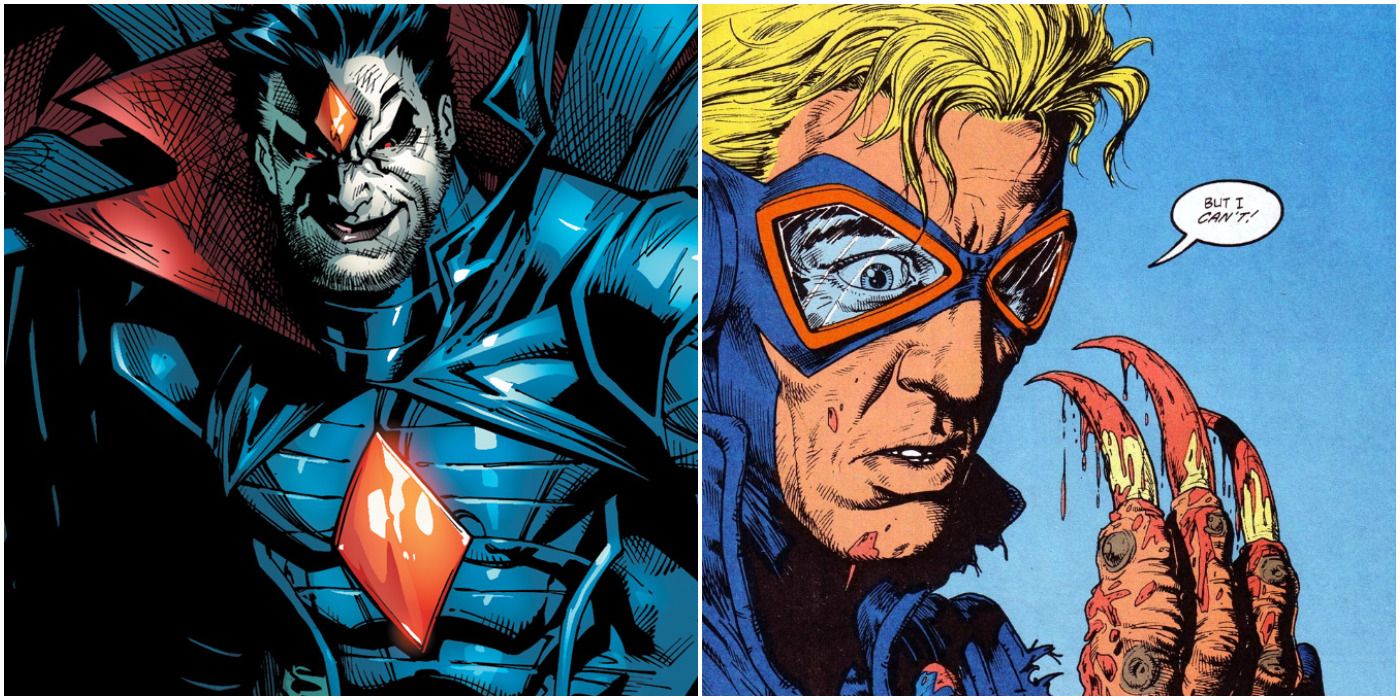The image consists of two comic book-style panels. The left panel features a sinister-looking character with black hair, a grimacing face, and a red diamond embedded in the center of his forehead. He wears a blue, ribbed armor-like suit adorned with a prominent red diamond on his chest, and has a large, dramatic collar that is red on the inside. The character's eyes are strikingly red, adding to his menacing appearance. Behind him, a blue cape can be partially seen.

The right panel depicts a blonde man wearing a blue and red uniform. His eyes are covered by blue and red goggles integrated into his suit, and he dons a blue jacket. The man is looking at his hand, from which yellow, blood-stained claws are emerging. The fingers of his hand appear to be brown with black markings. A speech bubble next to him emphasizes his words, "but I can't," with the word "can't" italicized. The background of his panel is light blue, contrasting with the darker tones of the left panel.